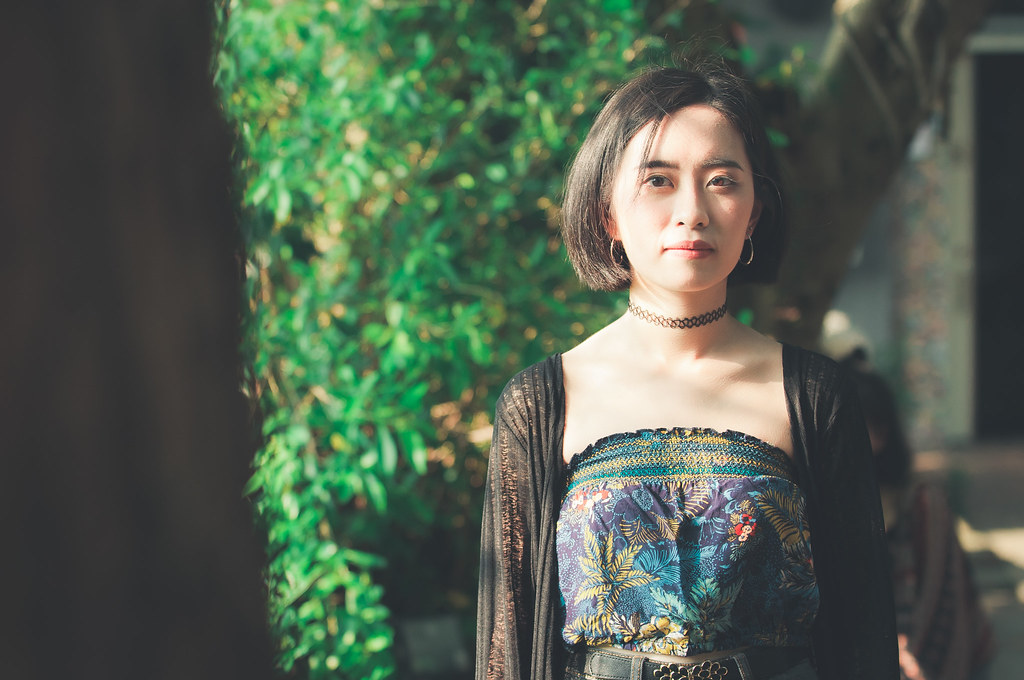The photograph features an Asian woman with a blunt bob haircut and dark, chin-length hair, styled with hoop earrings and heavy eyebrows. She wears a nudish color lipstick and a black choker necklace tightly around her neck. Her outfit consists of a vibrant strapless top adorned with an intricate design of illustrative plants, including shades of blue, green, yellow, and possibly some purple and red. Over her shoulders, there is a delicate, drapey, see-through shawl or jacket, likely black. Completing her look, she sports a belt at her waist. The background is slightly blurred, depicting lush greenery with a large branch extending to the side and a doorway visible to the right. The left side features an indistinct, blurry object that might be in the foreground. The setting appears to be outside, possibly in front of a tan or yellow building. The woman is approximately 30 years old.